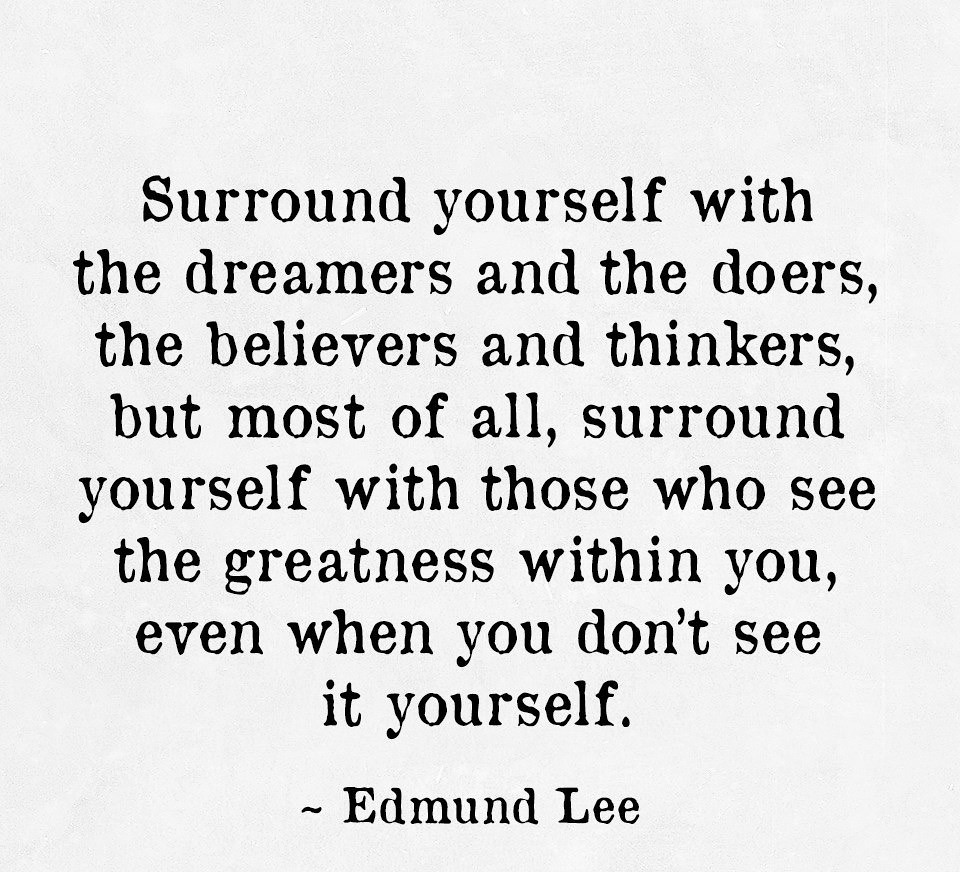The image features a motivational quote by Edmund Lee on a white square background, with centered black text resembling a typewriter font. The slightly blotchy text reads: "Surround yourself with the dreamers and the doers, the believers and the thinkers. But most of all, surround yourself with those who see the greatness within you, even when you don't see it yourself." The quote ends with a tilde and Edmund Lee's name. The background is plain with no additional design elements, focusing solely on the inspirational message.